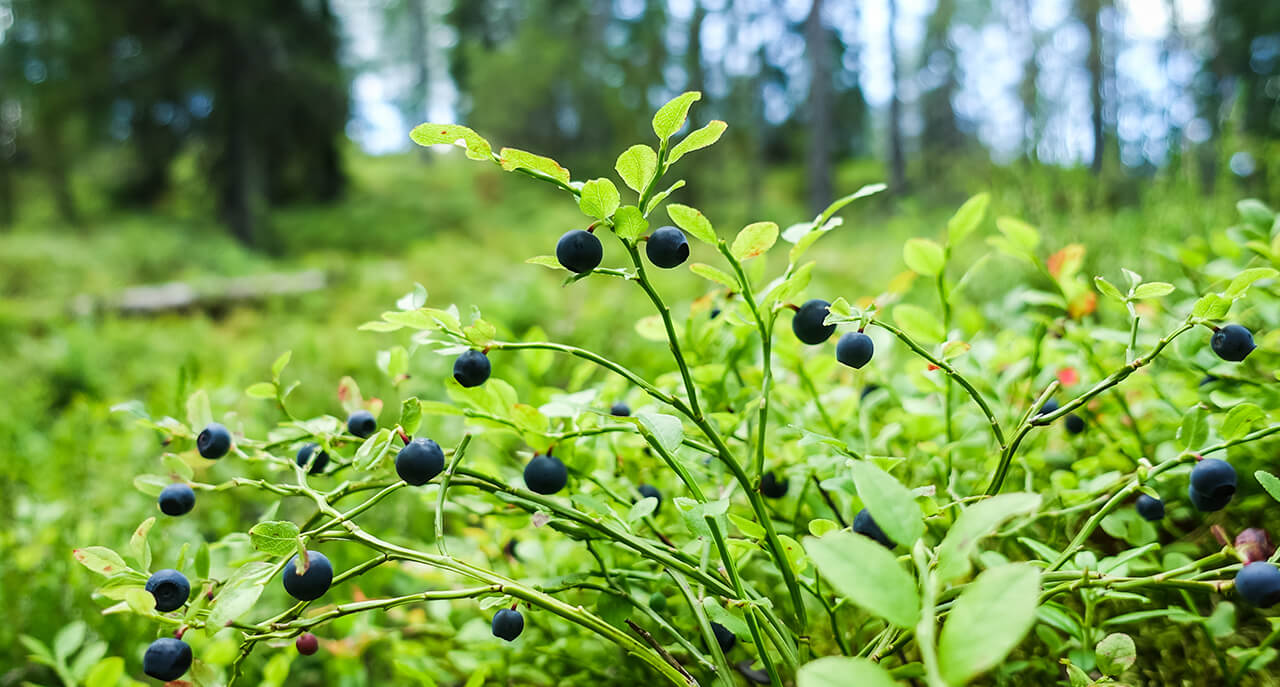This photograph showcases a cluster of blueberries hanging from slender plants, which display a range of green hues, from light to dark, and even some yellowish tones. The image captures the crisp and clear details of the foliage, with some leaves prominently featured in the foreground. The background reveals a patch of overgrown green grass, exhibiting various shades from light to dark, with some blades appearing dry. Beyond the grass, a line of trees stands, some more barren than others, with visible trunks and a soft, dappled sunlight filtering through the branches. The overall composition places the focus on the blueberries in the foreground, emphasizing the clarity and richness of the scene.